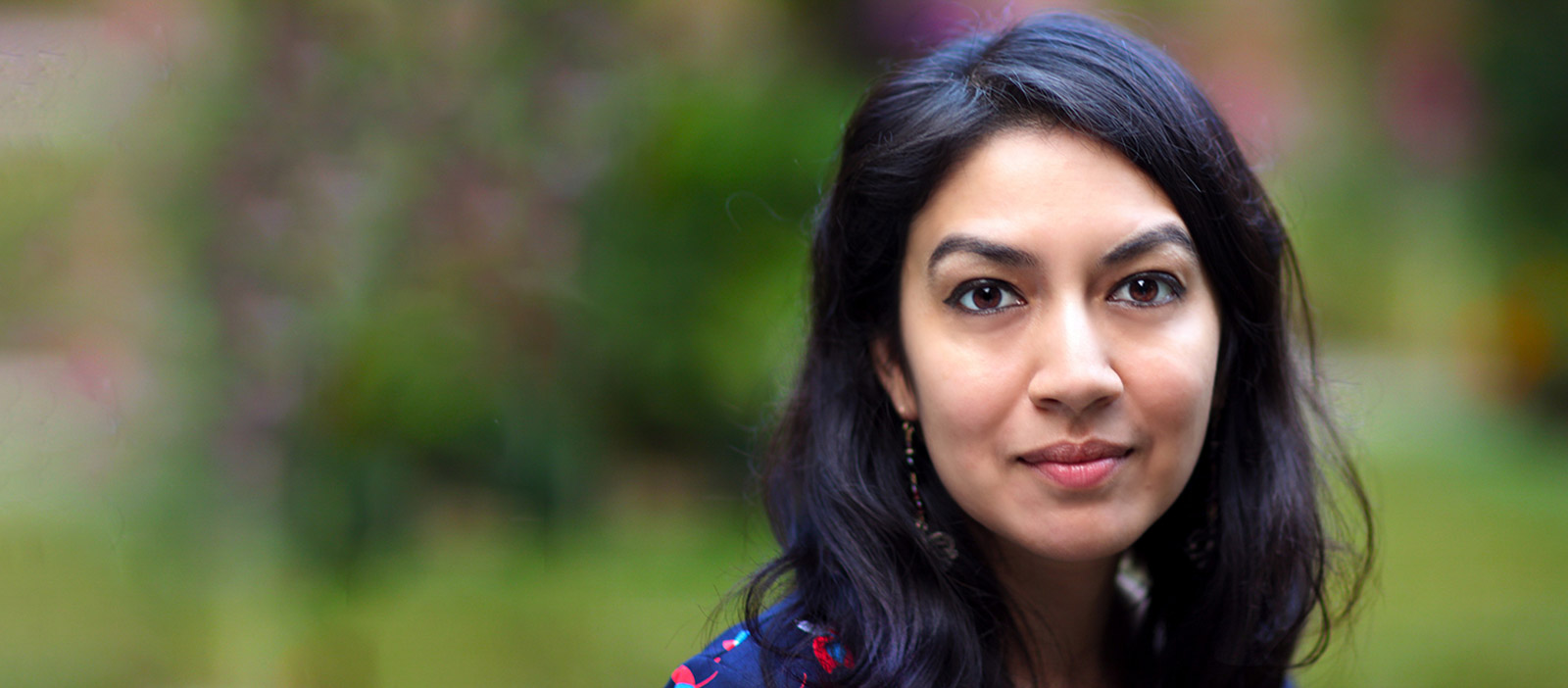This rectangular headshot features a striking woman situated to the right of the photograph. She has long, dark brown hair pulled away from her face and gazes directly at the camera with an intense, almost contemplative look. Her dark brown eyes are framed by arched eyebrows, and she wears minimal makeup, perhaps just a touch of pink lipstick. A notable mole rests underneath her right nostril. Her full lips and delicate eyeliner accentuate her expressive features. 

Long, dangling gold earrings adorn her ears, visible on the left side. She wears a dark blue shirt decorated with red floral patterns, from which only the left shoulder is visible due to the close-up nature of the shot. The background is intentionally out of focus, highlighting the greenery of trees and a subtle hint of pink, suggesting an outdoor setting. This composition centers on her face, capturing both her physical details and a glimpse into her thoughtful demeanor.